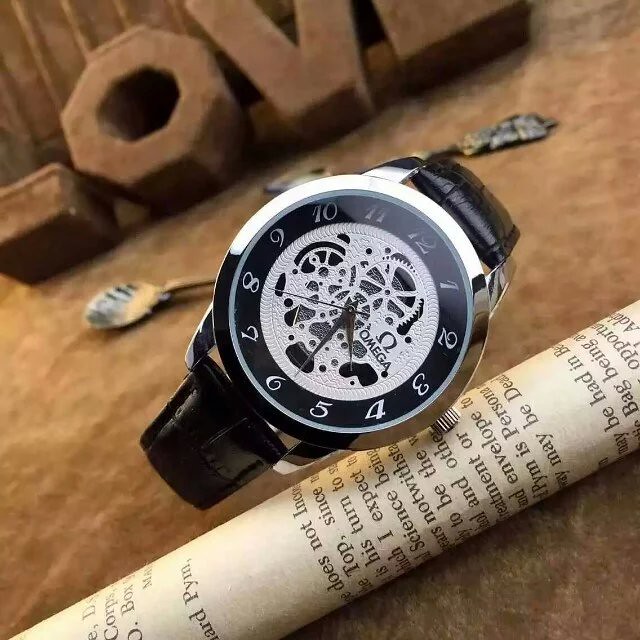A detailed description of this image would be:

A square photograph showcasing an elegant wristwatch prominently displayed at the center. The watch is positioned diagonally, stretching from the upper right to the lower left corner of the image. It rests against a rolled-up newspaper, which props it up at an angle towards the viewer. The black band contrasts strikingly with the silver body of the watch. The watch face features an outer black ring with white numerals, a white center revealing intricate gears, and sleek silver hour and minute hands. The distinguished Omega logo is clearly visible on the face. The background includes a slightly out-of-focus setting with a spoon and another utensil lying on what appears to be a wooden table, adding a touch of homeliness. Leaning against the backdrop wall, there's a blocky sign spelling out "LOVE," tying together a scene that balances sophistication and warmth.